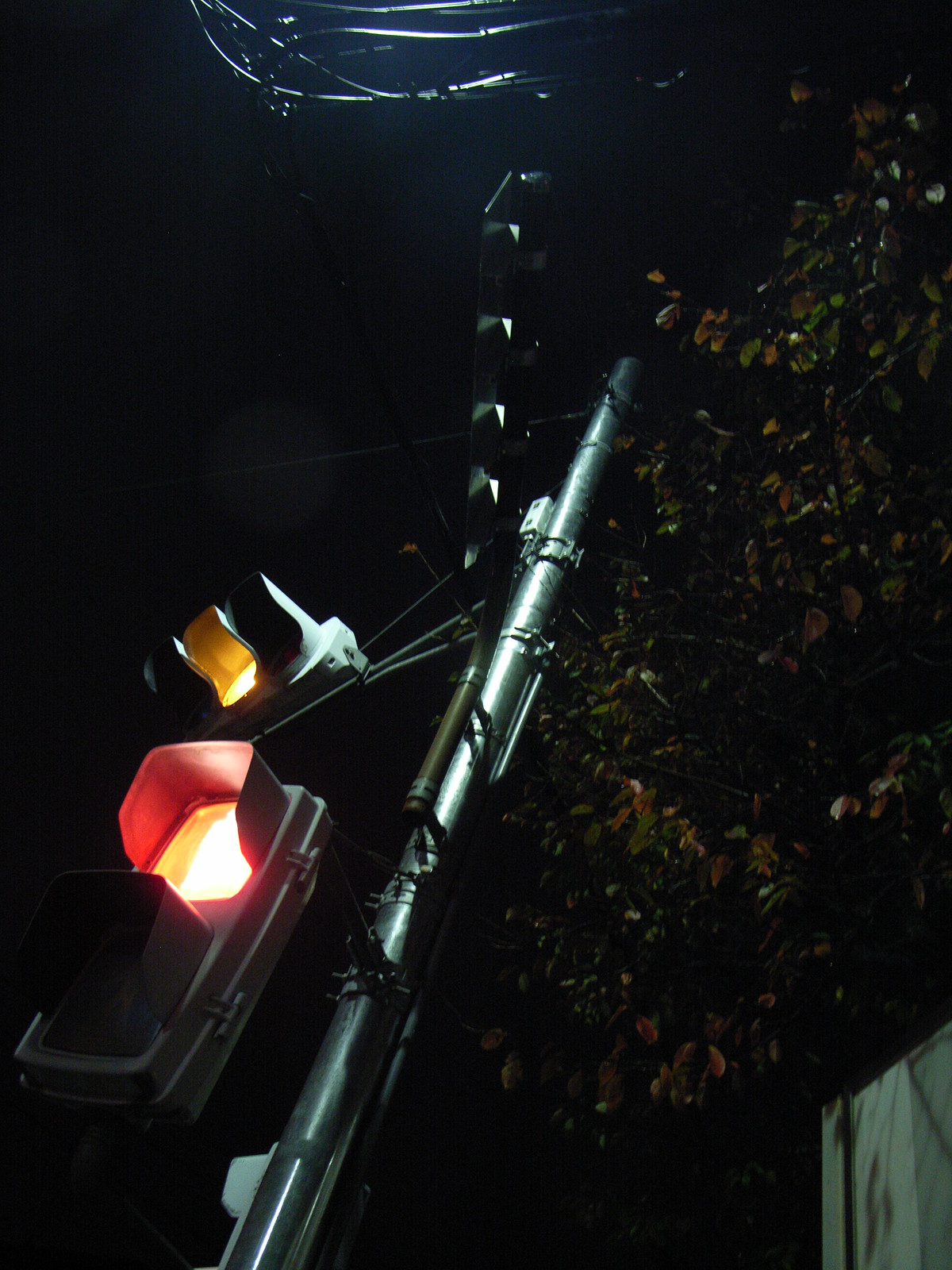A nighttime photograph captures a stoplight against a pitch-black sky with scarcely any stars visible. On the right side of the image, an imposing tree with dark-colored leaves partially envelops the stoplight, hinting at a late summer or early autumn setting. Beneath the tree, the faint outline of a white fence or shed peeks through the darkness. The stoplight, mounted on a substantial metal pole that extends high into the tree's canopy, prominently displays a yellow light indicating caution and a red light signaling stop. The lights seem to be arranged independently, one above the other, rather than as part of a single, cohesive unit.